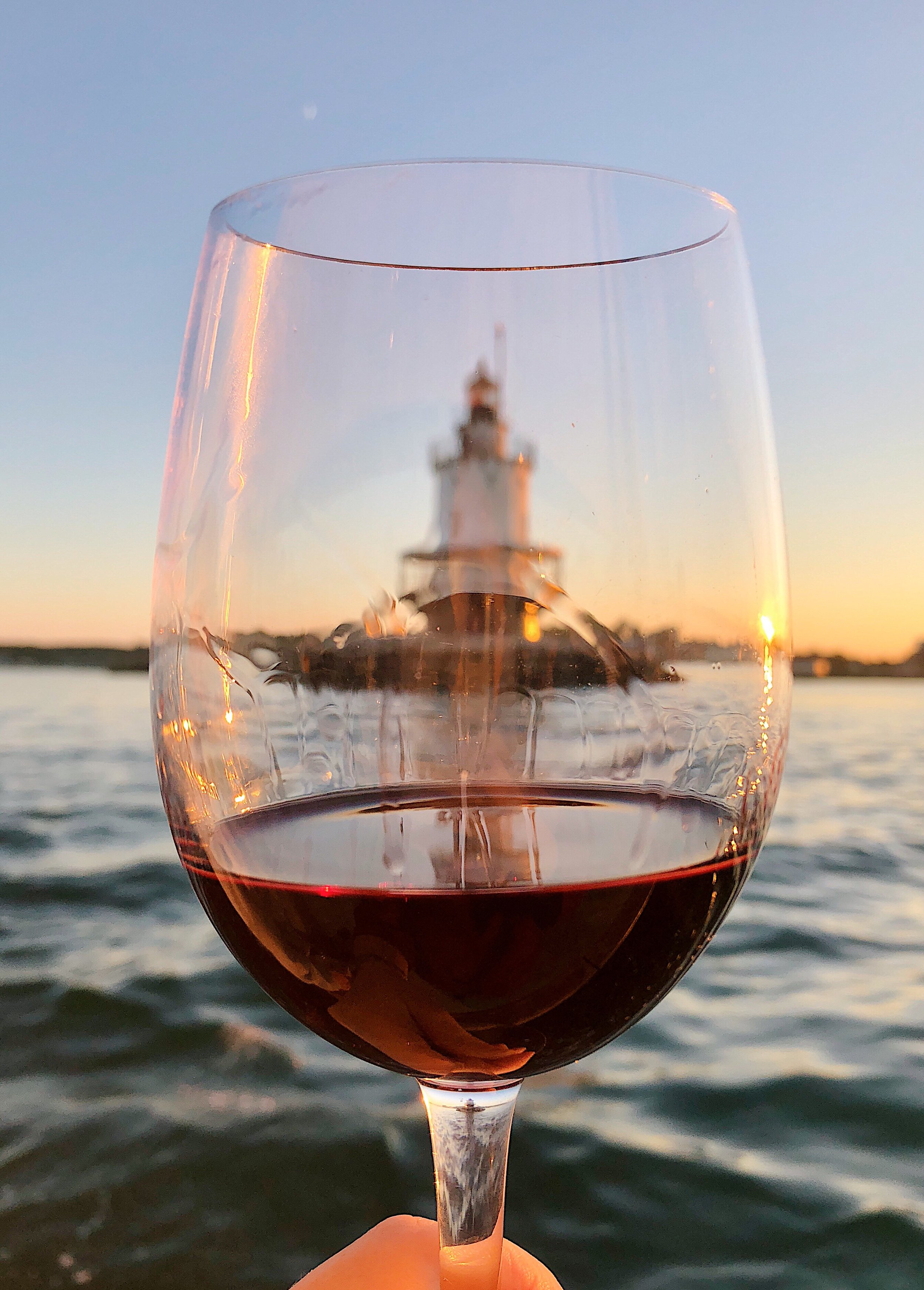In this photo, a wine glass dominates the foreground, taking up most of the frame and sharply in focus. The glass is filled a quarter of the way with a rich red wine, which has a brownish or maroon hue. Intriguingly, there are two pepper-like objects floating at the bottom of the glass. A hand is evident at the bottom of the photo, grasping the wine glass by the stem, with the top of a knuckle just visible. The background offers a serene vista of open water, likely an ocean, serving as the mid-ground. Through the glass and beyond, a blurred white structure with a pointed top—almost certainly a lighthouse—can be seen. The sky above transitions from a pinkish hue at the horizon, indicative of a sunrise or sunset, to a clearer blue sky, completing the tranquil atmosphere of the scene.